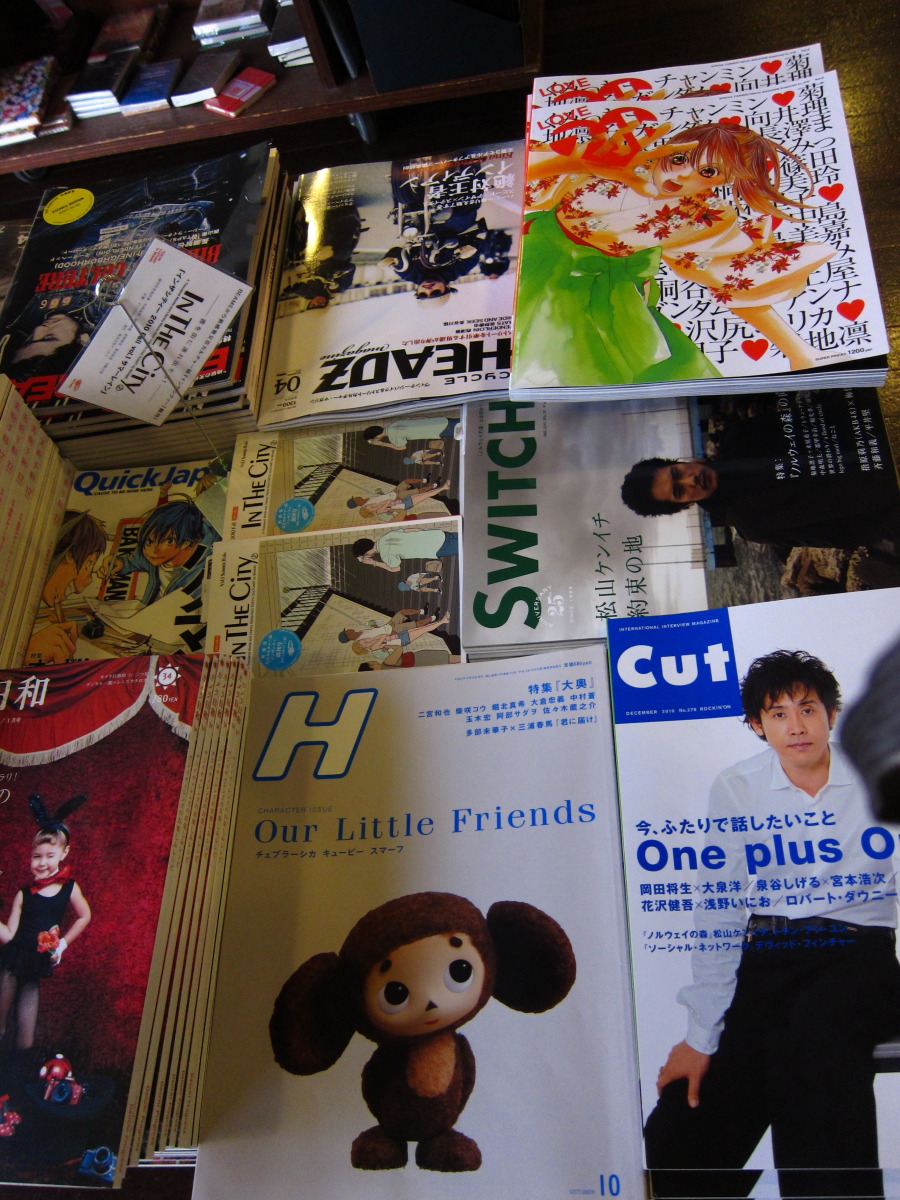A vibrant and colorful photograph captures a tabletop display in what appears to be a store setting, showcasing an eclectic assortment of magazines in both English and Japanese. The magazines are arranged into neat piles across the desk, with some titles prominently featured. In the foreground, one magazine titled "Our Little Friends" displays an endearing claymation-style character resembling a baby teddy bear. Another magazine, "Cut," seems to cater to men's hairstyles, as it features a man modeling his hair on the cover. The table also holds a magazine called "Switch" and another named "In the City." One magazine features an anime figure wearing a green dress adorned with red flowers, reaching out for something red. Scattered among the magazines are smaller items that appear to be matchbooks or notebooks, suggesting that this display is from a shop. In the background, a couple of shelves add to the commercial ambiance, holding more booklets or possibly small Bibles. The scene is devoid of people, except for those on the magazine covers, emphasizing the array of publications spread before the viewer.